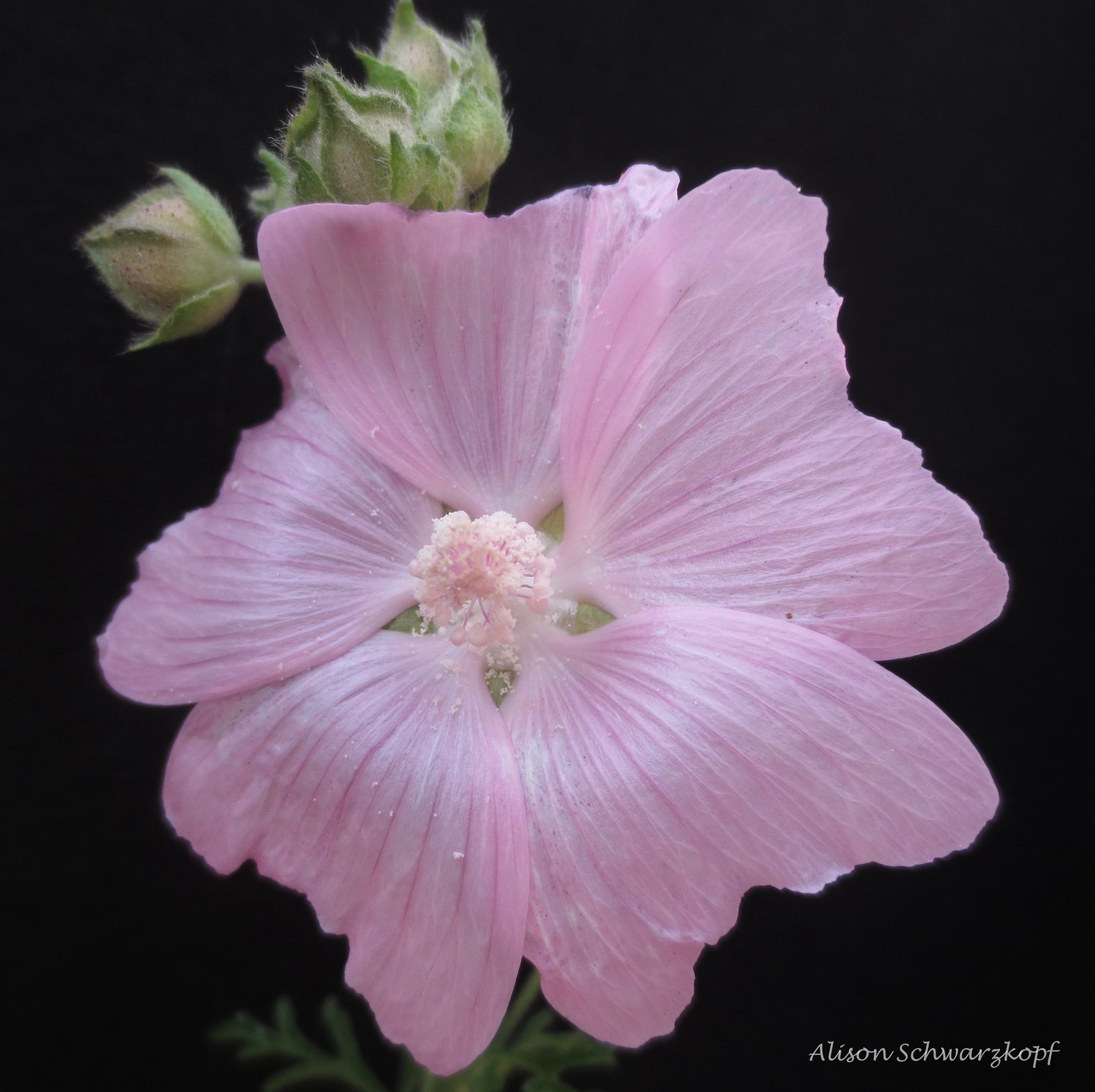This detailed photograph features a single, striking flower against a completely black background. The prominent bloom has delicate light pink petals that are fan or whale's tail-shaped and cover the majority of the image. The center of the flower showcases a light pink, fluffy structure. Surrounding the flower's center are five green leaves, adding a contrasting splash of color. The flower's green stem, adorned with small needles, ascends from the bottom of the frame. Above and slightly behind the main bloom are three green, fuzzy buds that have yet to open. In the bottom right-hand corner of the image, the name "Allison Schwarzkopf" is elegantly inscribed in white cursive, likely identifying the photographer.